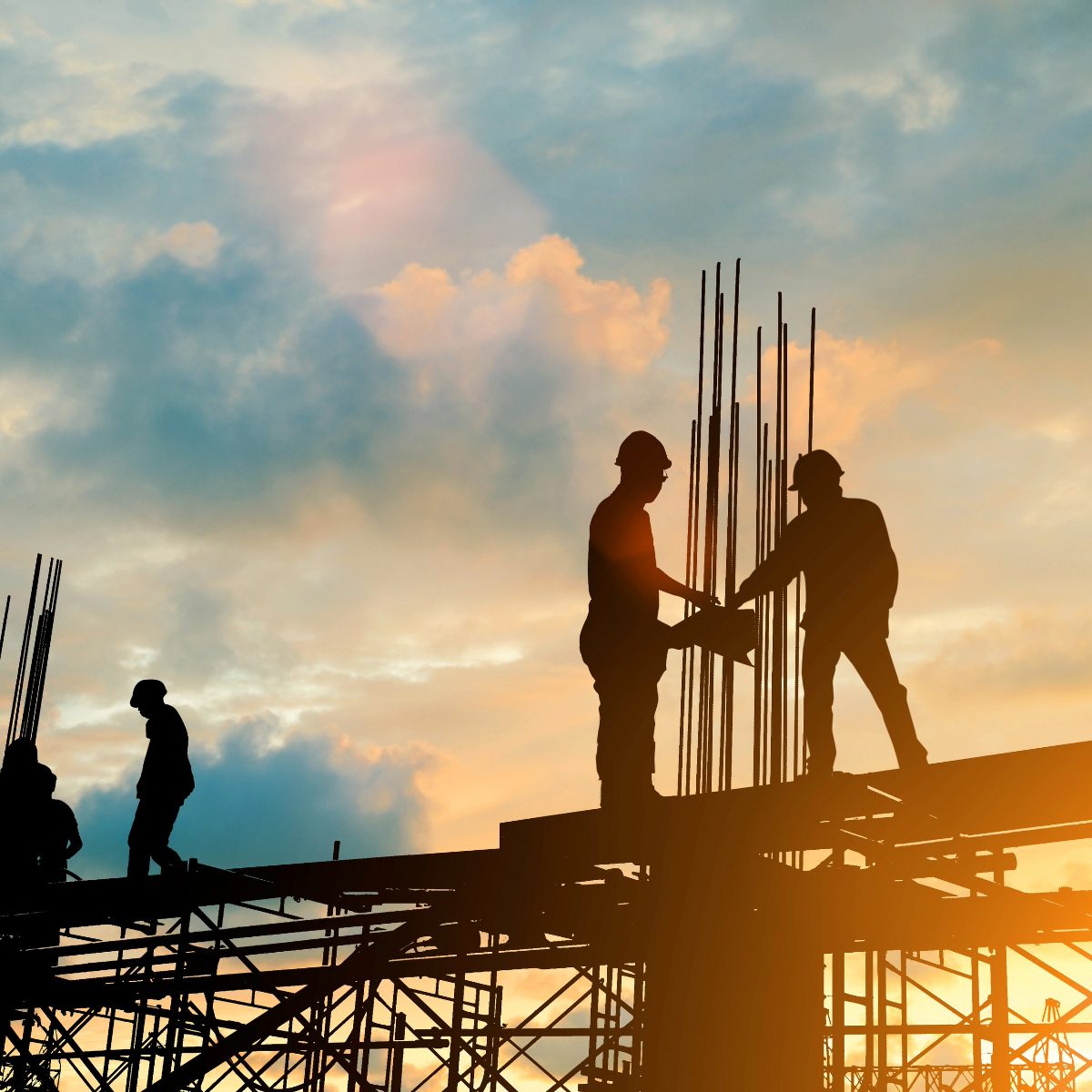This image captures a striking scene of a construction site during sunset in portrait orientation. The photo, characterized by its representational realism, depicts several construction workers donned in hard hats, silhouetted against the vibrant sky. The sun is setting toward the bottom right, creating a bright haze that casts dramatic shadows over the entire scene, rendering the workers as dark figures. 

Five construction workers are visible, but only their shapes can be discerned due to the intense backlighting. Two men on the right side of the image appear to be examining a piece of paper, likely construction plans, on top of a steel platform. Behind them rises a network of tall, vertical metal beams and scaffolding. To the left, additional workers and structural elements populate the scene, all enveloped by a complex metal framework spanning the bottom portion of the photograph. The sky above them is a striking mix of blues, pinks, and golden hues with scattered clouds tinted by the setting sun, adding depth and atmosphere to this industrial tableau.